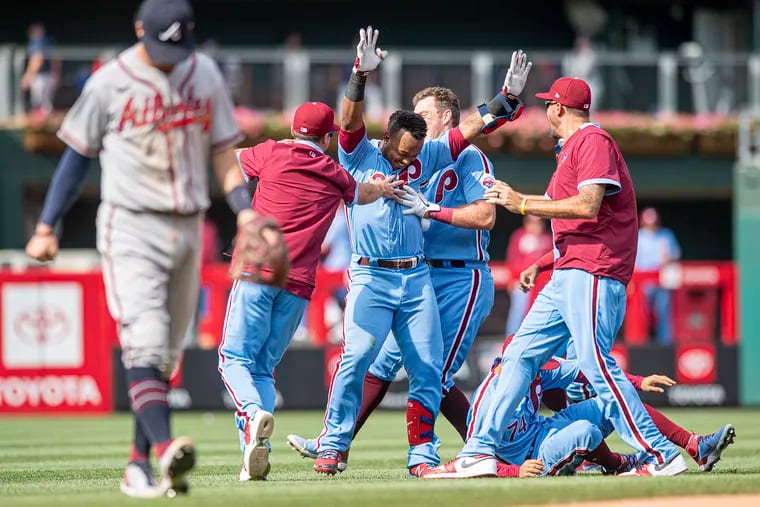In this vibrant daytime photograph of a baseball game, a group of players are captured celebrating exuberantly on a lush green field adorned with red, white, and black banners in the background. At the center of the image, a jubilant player stands with both hands raised high, smiling broadly. He is clad in a powder blue jersey with red lettering, accompanied by light blue pants featuring red stripes, and wears a brace on his left leg. Surrounding him are teammates and coaches dressed in matching powder blue uniforms with red accents. Two coaches in red shirts and light blue pants with red stripes stand out, one of whom sports a white glove on his left hand. Additionally, there's a player on the ground, having seemingly fallen in the midst of the celebration, and another walking away on the left, wearing a dark blue outfit with indistinct red lettering. The players all sport coordinated red cleats, belts, and socks, contributing to a cohesive and spirited team appearance.